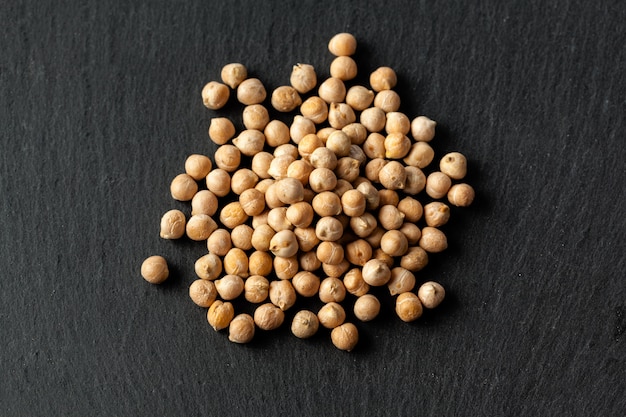This color photograph captures an overhead view of a tabletop surface adorned with a collection of approximately 75 to 100 dried chickpeas. These chickpeas are varied in hues, ranging from pale beige to light brown and yellow, and exhibit a mix of smooth and slightly wrinkled textures. Each of these legumes is characterized by a round shape tapering to a pointed tip. They are loosely grouped in the center of the dark gray background, which features vertical white striations suggestive of a marble pattern, and tiny white specks are visible, especially on the right side of the image. The surface could be a type of dark marble or a tablecloth, and the overall setting hints at preparation for a meal, possibly a healthy, spiced South Asian dish.